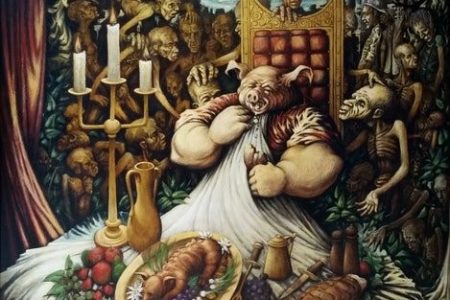This color painting is a detailed and thought-provoking depiction of gluttony. The landscape-oriented image portrays a grotesque human-pig hybrid seated to the right of the center in an opulent golden throne-back chair with a red quilted cushion. The pig, with food dribbling from its mouth, has human-like hands and wears a long white tablecloth as a bib, cinched at the neck. The lavish spread before it includes a platter with another pig, grapes, fresh fruit, a gold jug, and a salt and pepper shaker. There's also a tall three-candled candelabra on the left side and a red curtain framing the scene. Surrounding the throne are menacing skeletal-demon figures with big heads, jutting jaws, and wide noses, standing as though tempting or bearing witness to the pig's debauchery. The background and these figures add a haunting air, emphasizing the artwork's underlying message of excess and indulgence.